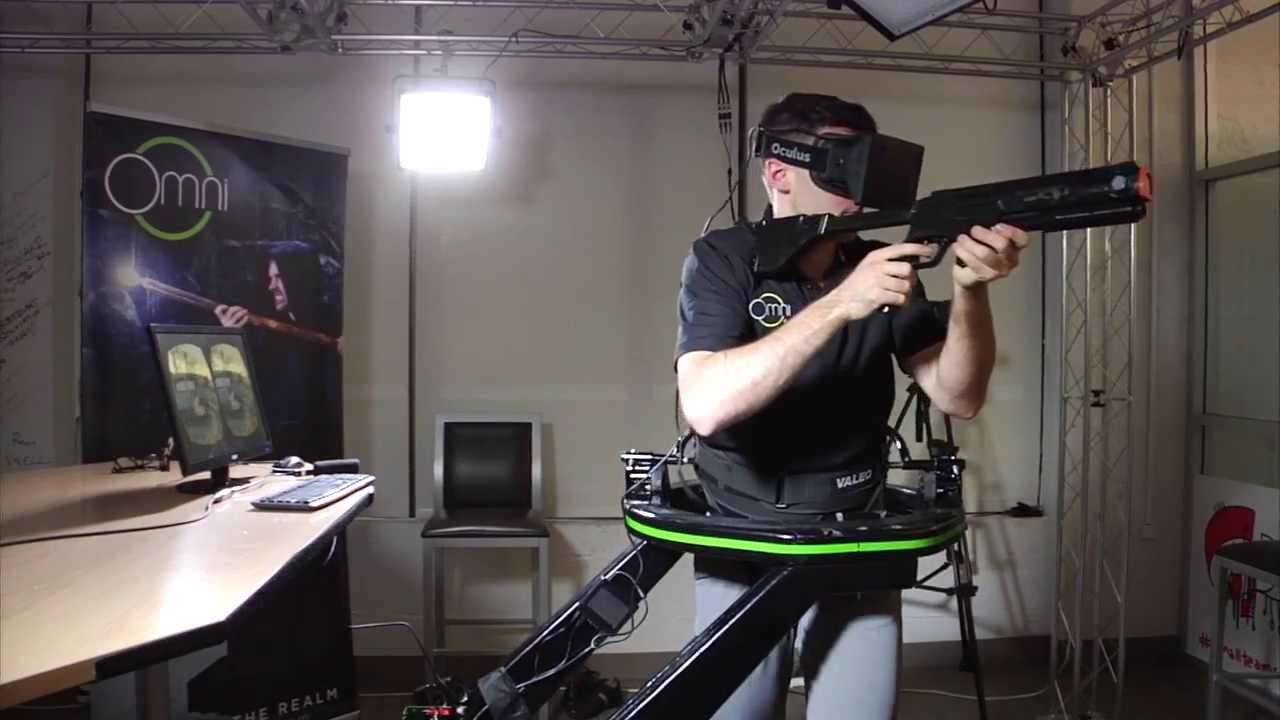The image depicts a light-skinned man with short brown hair, wearing a black short-sleeved shirt and light blue jeans, fully immersed in a virtual reality experience. He dons OCULUS virtual reality glasses, which are securely fastened with a strap around his head. Emblazoned on the left side of his chest is a circular emblem with the text "Omni," and his belt is labeled "VALEO." The man is gripping a toy rifle in both hands, with the butt of the gun pressed against his shoulder, suggesting he is engaged in a shooting game. He is attached to a sophisticated apparatus encircling his waist, designed to keep him stationary while he plays. The contraption includes two black metal supports extending to the lower left corner of the scene. The room itself is bright, except for the left side which features a poster for "Omni," possibly referencing a wizard game. A desk with a monitor and keyboard is also visible in the bottom left corner, enhancing the high-tech atmosphere of the setting.